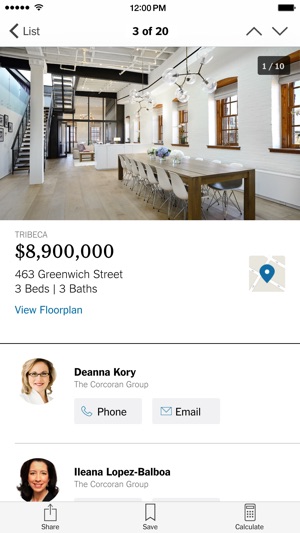For sale: Luxury loft at 463 Greenwich Street, Tribeca, priced at $8,900,000. This expansive residence offers three spacious bedrooms and three modern bathrooms. The listing highlights a new floor plan in the esteemed ACWA building. Represented by Dina Corey of The Corcoran Group, and Alina Lopez-Balboa, also of The Corcoran Group. 

The featured image showcases an open-concept living space typical of loft designs. A long wooden dining table, seating 12, is prominently placed in the room. The space is accented by large wood-trimmed windows that flood the area with natural light. The interior boasts a hardwood floor and a structural pillar, adding to the loft's industrial charm. A staircase, with multiple steps, leads to the upper level. Adjacent to the dining area, separated by a half wall, is a cozy living room space. Contact The Corcoran Group for more details on this stunning property in one of New York City's most sought-after neighborhoods.